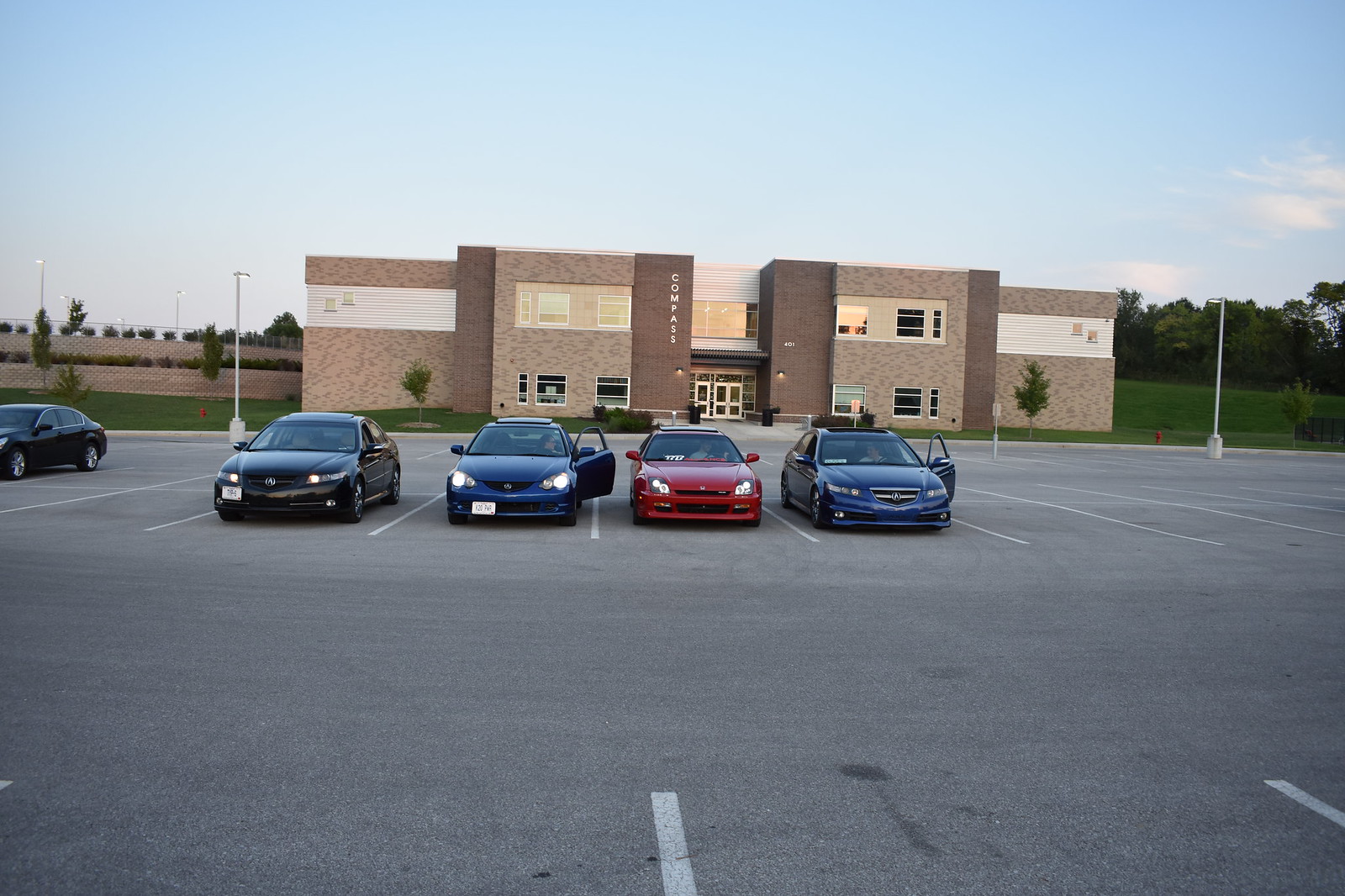The photograph captures an outdoor scene under a clear blue sky with faint wisps of clouds. Dominating the background is a two-story brown building with the word "COMPASS" prominently displayed in white capital letters, accompanied by the number "401" near the entrance. The building features a mix of dark brown and sand-colored face brick textures, with horizontal white stripes and a pair of glass doors framed in white.

In the foreground stretches a large parking lot with clearly marked parking spaces. Centered in the image is a row of four parked cars, all facing forward. From left to right, the vehicles are a black car, a dark blue car with its driver's door open, a red car, and another dark blue car, also with its driver's door open. Notably, the first three cars have their headlights switched on, while the last car does not. There are grass patches on either side of the building, enhancing the natural ambiance. A silver street light with a white lamp is visible on the far left, and additional pole lights in the distant background suggest that it is dusk.